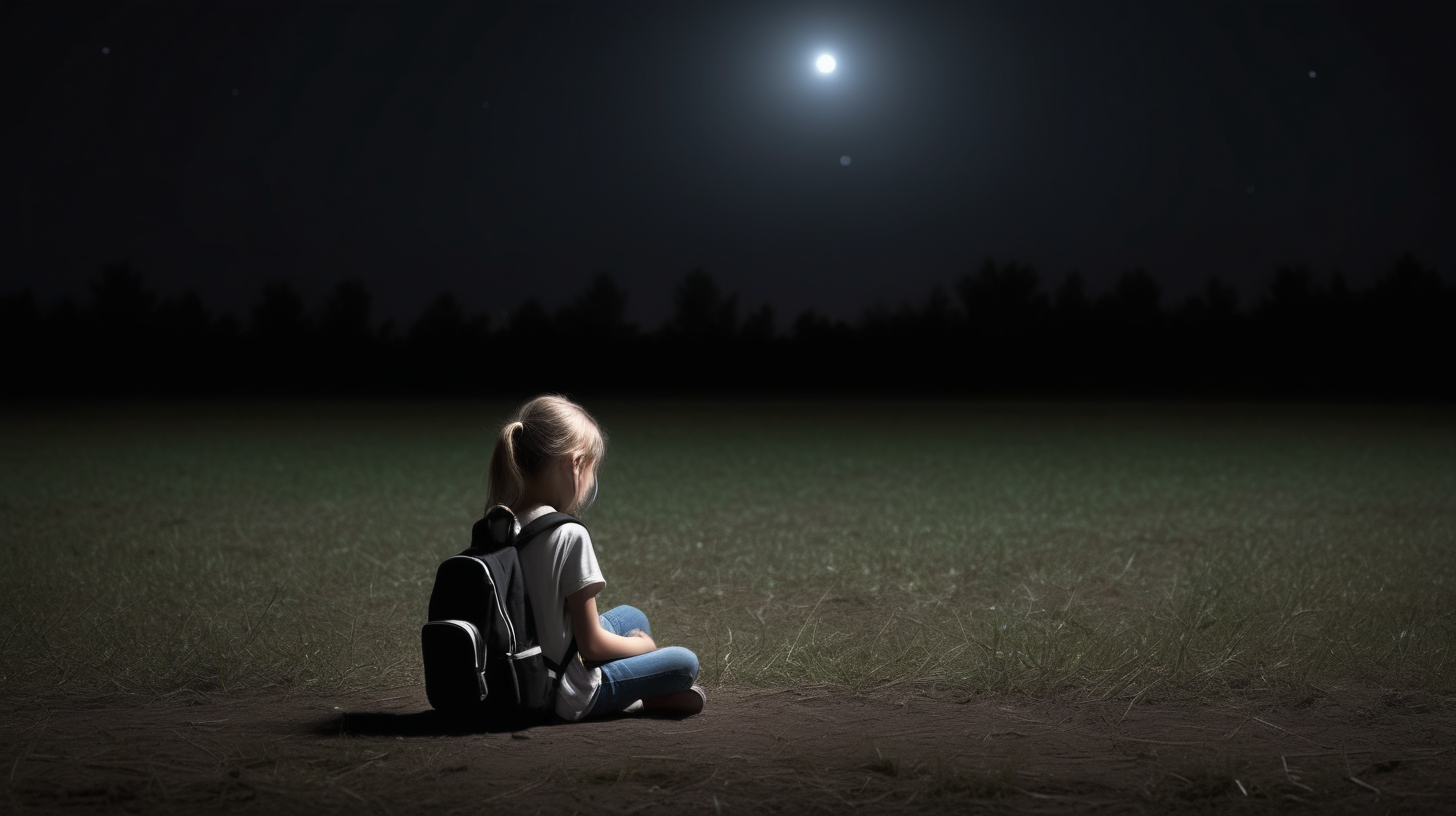In a serene nighttime photograph, a young blonde girl, around 8 years old, sits cross-legged on the ground wearing a light green t-shirt and jeans, with a black and gray backpack on her back. She faces away from the camera, calmly absorbing the moonlit scene before her. The backdrop features a sparse field with patches of greenish grass and dirt immediately surrounding her, while the blurred grass in the distance merges with silhouettes of trees. Above in the black sky, the main source of light is a bright moon, complemented by a faint, distant shape of another light. The subtle illumination from the moon casts a gentle spotlight on the girl, adding an ethereal quality to the tranquil scene.